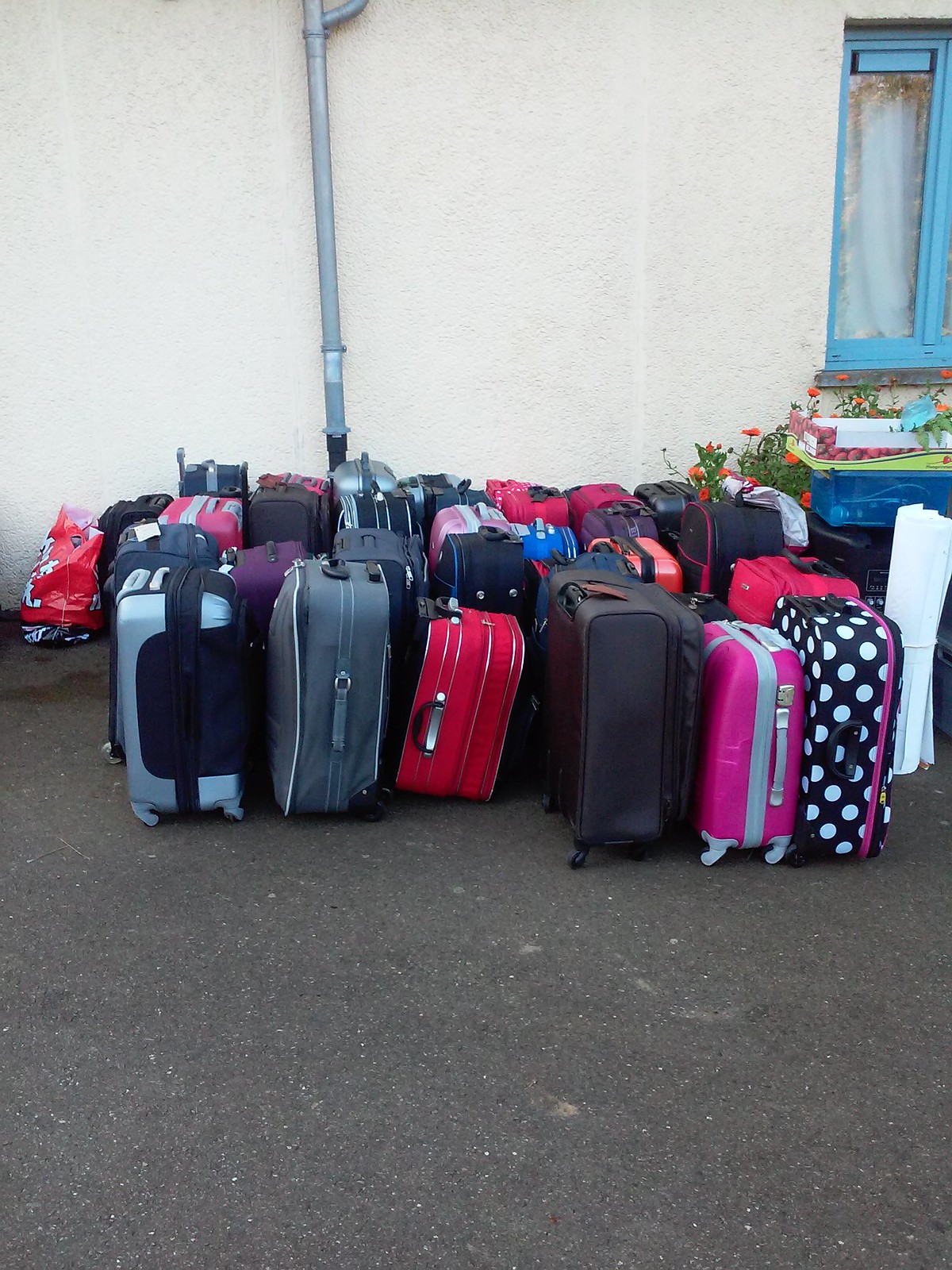This vertical, realistic photograph captures an outdoor scene in front of a beige stucco house. At the center of the image, a stainless steel metallic pipe ascends vertically, flanked on the right by a blue-framed window adorned with white curtains. Below the window, a wooden flower box cradles red flowers. The ground, composed of dark brown dirt or fine gravel, hosts an array of approximately 20 to 30 roll-on suitcases, suggesting a well-organized collection. 

The suitcases, mostly rectangular and uniform in size, display a spectrum of colors including black, gray, red, pink, blue, yellow, purple, and one with white polka dots. They are all neatly lined up side-by-side, standing on their wheels, with no visible text or branding. The setting exudes an impression of a slightly worn but charming household, possibly indicative of a family preparing for a trip or a storage scenario. The arrangement of the suitcases suggests a moment of organized chaos amidst the quiet backdrop of the house.